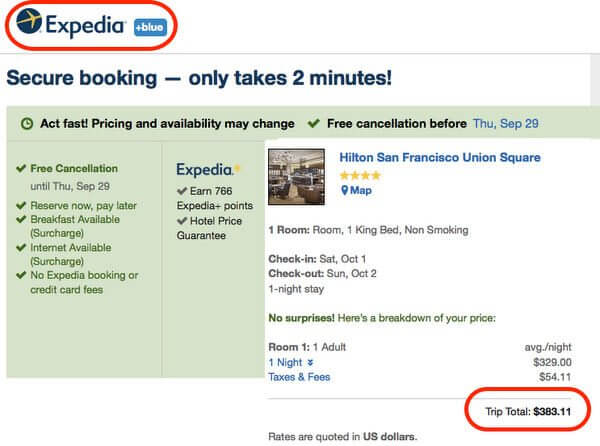Title: Detailed Overview of Expedia Booking Screen

Description: 

This image is a screen capture from the Expedia website. At the top, there is a prominent red-orange box highlighting the Expedia logo, next to which is a navy and gold airplane icon signifying the travel theme of the site. To the right, a blue box contains white text, detailing the site's blue-themed interface.

Further down, in navy text, a message assures users that secure booking takes only two minutes. The background then transitions to green, featuring a black text alert with small green icons, stating: "Act fast, pricing and availability may change," followed by a blue date marking free cancellation until Thursday, September 29.

Continuing down, there are more user benefits listed with green, gray, and navy fonts: "Free cancellation until THU September 29," and "Reserve now, pay later," with green check marks. Additional features include "Breakfast available (surcharge)," "Internet available (surcharge)," and "No Expedia booking or credit card fees." A section in navy text notes: "Earn 766 Expedia points," alongside "Hotel price guarantee."

On a white background, detailed information about the hotel is presented. In blue text, it identifies the hotel as "Hilton San Francisco, Union Square," rated four stars with a map icon indicating the location. An interior view of the hotel's lobby is shown.

The booking details specify: "One room, one king bed, non-smoking," with check-in on Saturday, October 1st, and check-out on Sunday, October 2nd, for a one-night stay. A reassuring green text states: "No surprises: Here's a breakdown of your price," followed by a mix of gray and blue fonts that itemize the cost as follows: Room for 1 adult at $329, with taxes and fees amounting to $54.11, culminating in a trip total of $383.11, highlighted within a red box. Lastly, it's indicated that all rates are quoted in U.S. dollars.